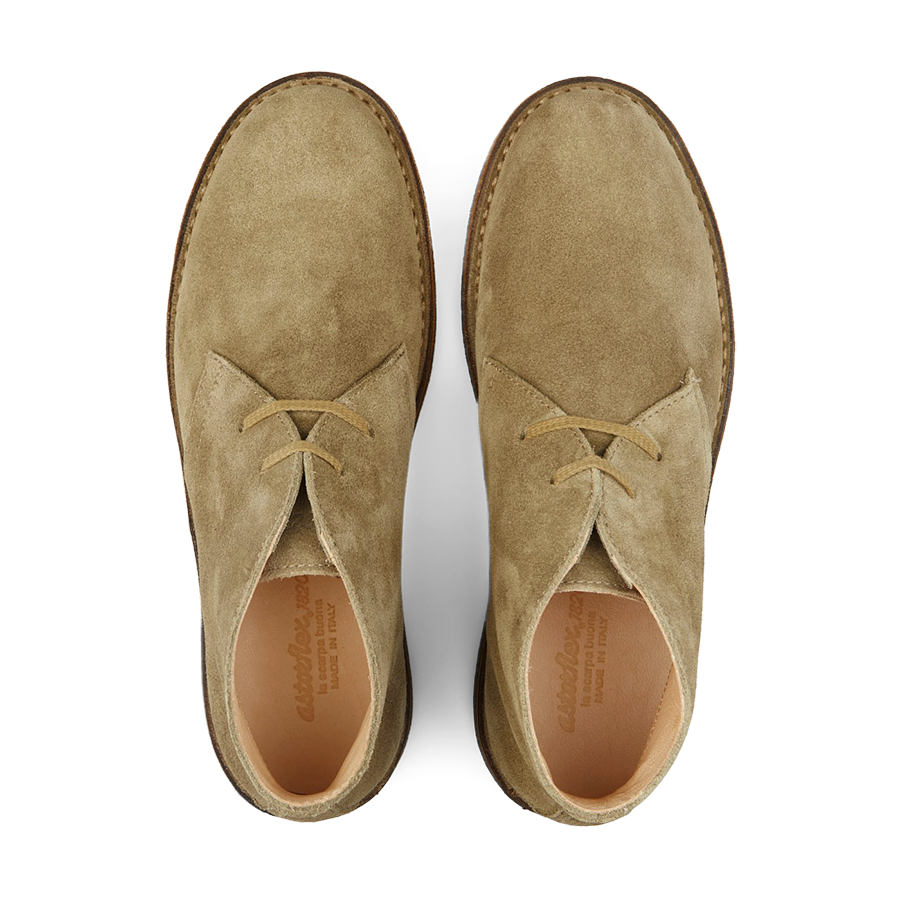This is a detailed photograph taken from above of a pair of light brown leather or suede moccasins. Made in Italy, these shoes exhibit fine craftsmanship evident in the intricate stitching around the outer edges and the sleek design of their thin, flat brown soles. Each shoe features two shoelaces threaded through four holes, with the laces wrapped twice around each shoe for added detail. The insides are a vivid pink with an orange hue, inscribed with cursive Italian words, including "made in Italy" and "buona," though the full text is difficult to decipher. The shoes are meticulously positioned with their toes at the top of the frame, presenting a clear view of their elegant silhouette and refined leather texture.